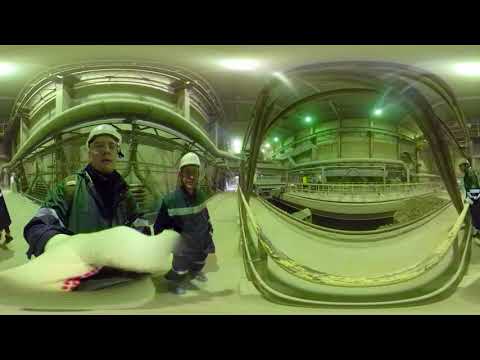In this image, two middle-aged men are seen working inside a large industrial factory specializing in conductive valves. Both men are outfitted in white hard hats and blue industrial overcoats with reflective strips on the sleeves, adding a layer of safety and visibility in this protective gear. The image, captured with a 360-degree panoramic fisheye lens, has a distinctive, slightly distorted effect that curves straight lines towards the center, giving the impression of peering through a fishbowl.

The scene is bathed in green-tinted light, possibly due to the unique camera settings or filters, casting an almost surreal atmosphere. The two primary subjects are looking directly at the camera, with one man appearing to reach out towards it, indicating a curiosity or interaction with the camera. In the background, another man leans over a yellow railing, which also appears green because of the lighting, gazing down into what seems to be a large pit filled with machinery, tubes, and rocks—a common sight in industrial settings. This detailed snapshot of a bustling and technical workplace offers an intriguing and dynamic glimpse into a productive day at the factory.